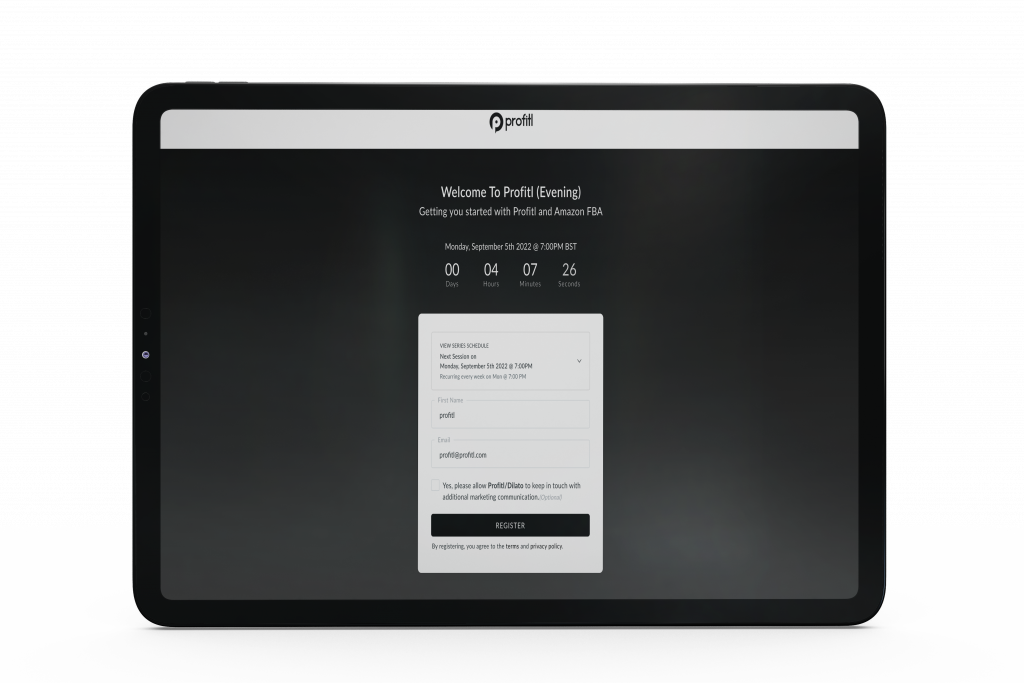The image depicts a screenshot or photograph of a tablet screen. The screen has a distinct black border with a whitish-gray camera notch on the left side. The top of the screen features a white header strip that spans across the display, showcasing a logo consisting of a circle with a "P" cut into it. The "P" is white, blending seamlessly with the white background. Adjacent to the logo, the text "Prophet" is displayed in black.

Below the header, the background transitions to black. Prominently displayed in large white text at the top is the greeting, "Welcome to Prophety," followed by "evening" in parentheses. Directly beneath this, in smaller white text, are the words "Getting you started with Prophety and Amazon FBA." The event date and time are also listed in white text, stating: "Monday, September 5th, 2022 at 7pm BST."

The screen further includes a countdown timer indicating time remaining: "00 days, 04 hours, 07 minutes, and 26 seconds." Toward the bottom of the display is a white box containing registration information, although the specifics are not legible. The box features a prominent black button at the bottom, with "Register" written on it in white text.